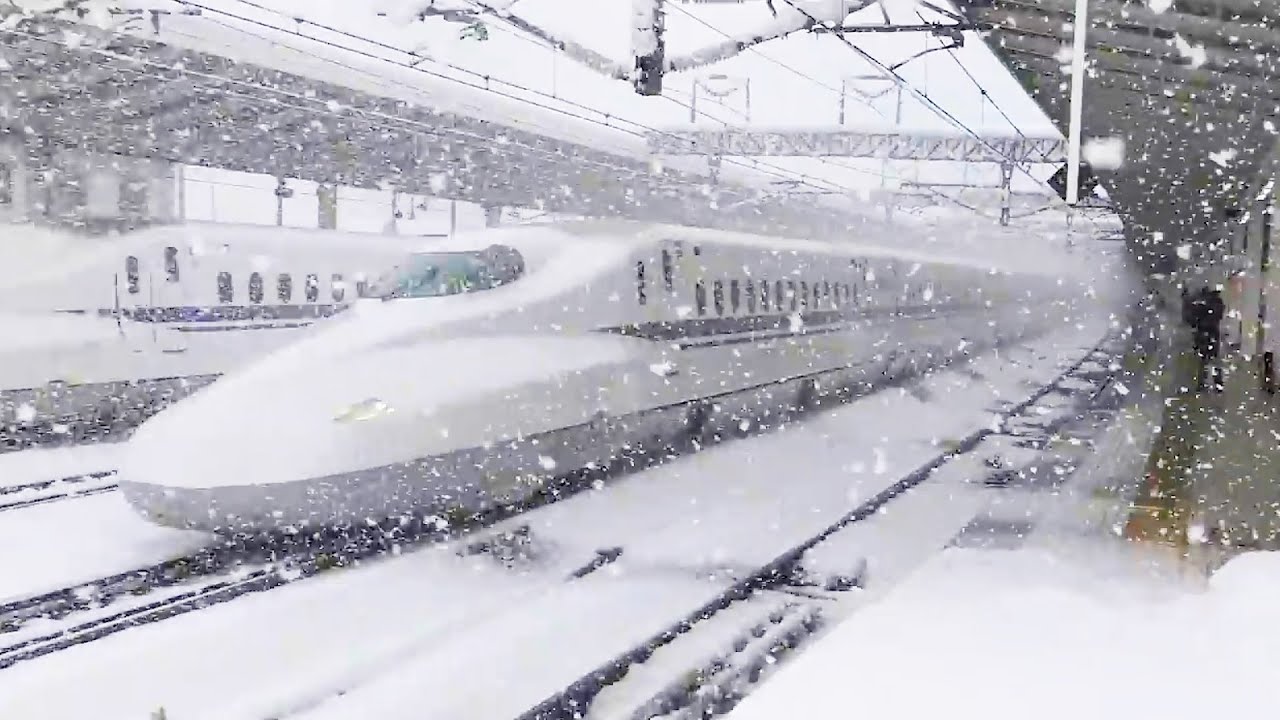In this heavily snow-laden photograph, a scene from a snowstorm is captured in color, showcasing a modern bullet train, perhaps in Japan, either pulling into or out of a station. This sleek, white train, with gray trim on the bottom and a blue stripe down its windows, dominates the image. The snowy backdrop blurs some of the features, but visible details include the snow-covered tracks and the canopy on the right, indicating a boarding area. A person dressed in black stands on the platform, barely discernible through the heavy snowfall of large flakes. Another train appears on the opposite side, its nose just visible, suggesting the presence of multiple tracks. The snow piled on the rafters and wires above enhances the wintry atmosphere, blending seamlessly with the train and the ground both blanketed in white.